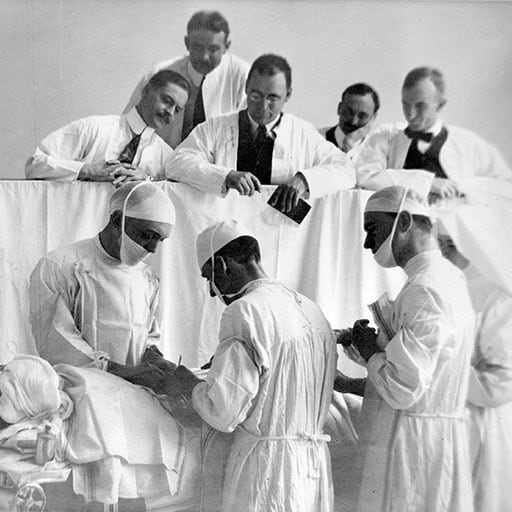This black and white photograph captures a detailed and intense scene of a surgical operation. In the foreground, three male surgeons, clad in white gowns, masks, and caps, are meticulously working on a patient covered with a white sheet. Standing to their right is a nun in a white frock, likely assisting or observing the procedure. Nearby, another man, also dressed in a white medical uniform, is closely watching the surgery unfold.

Elevated above the operating area, a group of five male doctors, identifiable by their white lab coats worn over suits, intently observe the procedure. They lean over a ledge draped with a white cloth, likely functioning as a viewing barrier. One of these observers, positioned at the front and wearing glasses, holds a notebook, possibly taking notes on the surgical process. All individuals in the photograph appear to be Caucasian.

The image conveys a sense of a medical training or evaluation session, with seasoned doctors overseeing and possibly instructing younger surgeons. The stark contrasts of the black and white photography emphasize the sterile and serious environment of the operating room.